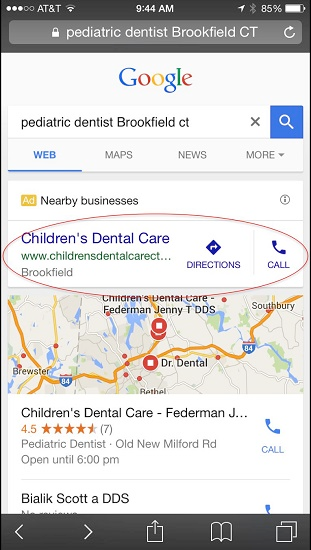The screenshot captures the display of a smartphone, featuring the Google search results for "Pediatric Dentist Brookfield CT."

At the very top of the screen, the status bar displays various symbols and indicators:
- On the top left, there are three white circles followed by two white circles, indicating signal strength.
- Next to the signal indicator, the network name "AT&T" is displayed, with the ampersand symbol.
- The center of the status bar shows the time, "9:44 AM."
- On the right side, icons for Bluetooth and the battery level are present, indicating 85% battery with a small portion still charging.

Below the status bar, a gray search bar is prominently featured, containing the text "Pediatric Dentist Brookfield CT" in white.

Directly beneath the search bar, the Google logo is displayed with the letters: "G" in blue, "o" in red, another "o" in yellow, "g" in blue, "l" in green, and "e" in red. Accompanying this is another search input box, this time with the earlier search phrase "Pediatric Dentist Brookfield CT" in black text. A blue box with a white magnifying glass icon is positioned for initiating a search.

Below the search functionalities, a horizontal menu shows search categories:
- "Web" highlighted in blue.
- "Maps," "News," and "More" in gray, with "More" having a dropdown arrow.

The next section starts with a white box containing a small yellow box marked "AD" in white, indicating an advertisement. Following this, the text "Nearby Businesses" is displayed in black.

Proceeding to the actual listings:
- The first result, in blue text, is "Children's Dental Care," with the green URL "www.ChildrenDentalCT.com" trailing off into ellipses.
- The word "Brookfield" is shown in gray beneath the URL, with "Directions" in blue to the right and "Call," circled in red, further to the right.

A map of the area displaying multiple pins for Pediatric Dentists in Brookfield, Connecticut, is visible below the first listing.

Under the map, the second listing includes:
- "Children's Dental Care-Fiedermann J" in black, accompanied by several rating stars.
- Below this, another entry, "Beliot Scott A. DDS" in black text, appears in the list.

This image provides a thorough depiction of a typical Google search result page for pediatric dentists in Brookfield, Connecticut, complete with search inputs, advertisement features, navigational links, contact options, and a geographic map for additional context.